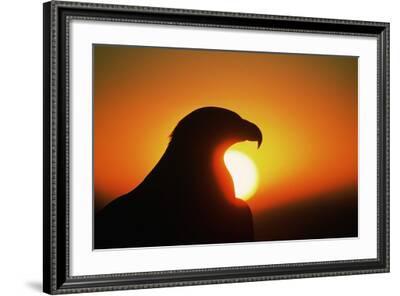This product photo showcases a framed photograph of a bird of prey, specifically an eagle or hawk, silhouetted by a vibrant sunset or sunrise. The bird is facing to the right-hand side, with its sharp, hooked beak prominently outlined against the backdrop of a low-horizon sun. The sun, partially visible, casts a bright glow highlighting the bird's head and shoulders, surrounded by a gradient sky that transitions from deep orange to yellow. The bird is rendered in a dark silhouette, emphasizing its powerful form against the colorful backdrop. The photograph itself is framed in a dark-colored frame with intricate beaded detailing around the edges, and a white matting surrounds the image. The entire scene, striking in its simplicity and contrast, is set against a plain white background, drawing attention to the dramatic composition within the frame.